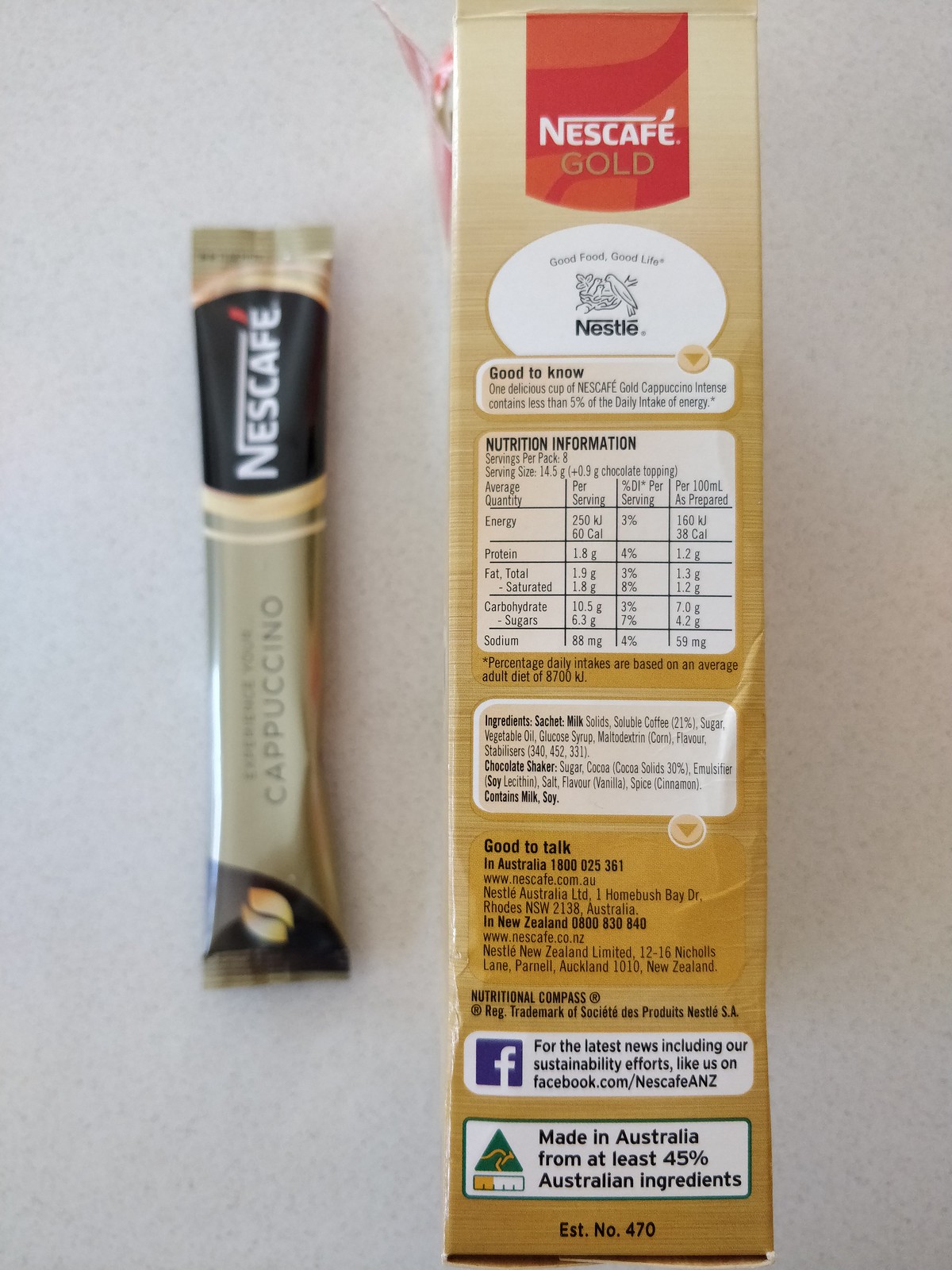The image features a Nescafé Gold Cappuccino sachet set on a sleek gray background. The sachet prominently displays the iconic Nescafé logo with an accentuated 'é' in red, encapsulated in a gold circle against a brown backdrop. The left corner of the sachet's gold packaging showcases a coffee bean design. 

Adjacent to the sachet, there is detailed text outlining the product's nutritional content per serving, including 60 kcals of energy, 1.8 grams of protein, 1.9 grams of fat, 1.8 grams of saturated fat, 10.5 grams of carbohydrates (6.3 grams of which are sugars), and 88 milligrams of sodium. These values contribute less than 5% of an average adult's daily intake based on a diet of 8,700 kilojoules.

The ingredients listed are comprehensive, consisting of milk solids, soluble coffee (21%), sugar, vegetable oil, glucose syrup, maltodextrin, corn flavor, and various stabilizers (E340, E452, E331). The accompanying chocolate shaker contains sugar, cocoa (with 30% cocoa solids), an emulsifier (soy lecithin), salt, vanilla flavor, and cinnamon spice. The product contains milk and soy allergens.

Additional information indicates customer service contacts for Australia (1-800-025-361, www.nescafé.com.au) and New Zealand (0-800-830-840, www.nescafé.co.nz), along with the respective addresses of Nestlé’s regional offices. The packaging also features a white label with the Facebook logo, encouraging consumers to follow the brand for updates on sustainability initiatives at facebook.com/NescaféANZ. 

Moreover, there is an emblem with a green border, inside which is a triangle with a kangaroo symbol and a ruler marked in gold, stating "Made in Australia from at least 45% Australian ingredients, EST.No.470."

This box set includes single-serve sachets of Nescafé Gold Cappuccino and a chocolate shaker, designed to provide a rich, flavorful coffee experience.